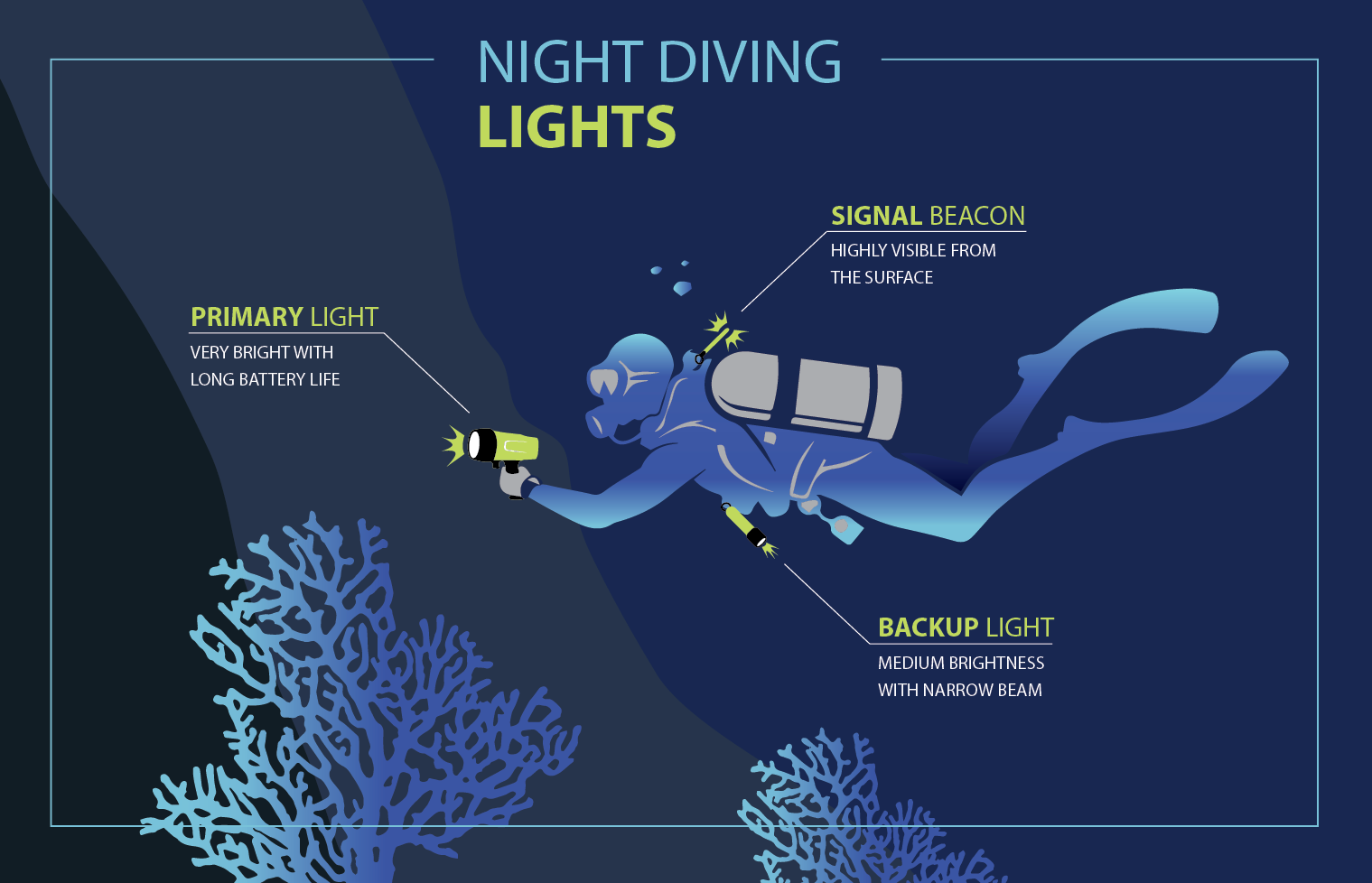This diagram is an informational illustration about night diving lights set against a dark blue background with gray and black accents. The entire image is framed with a thin light blue line that breaks at the top where the words "night diving" appear in the same color, followed by "lights" in bold yellow letters. 

In the foreground, the simple yet detailed illustration of a diver is shown in shades of blue, gray, and yellow. The diver, positioned swimming to the left, is equipped with a silver-trimmed scuba tank, goggles, a mouthpiece, fins, and a wetsuit. Three specifically labeled lights highlight essential gear for night diving. 

The diver's right hand holds a yellow and black flashlight labeled "primary light," described as very bright with a long battery life. On the diver's gear near the back of the neck is a "signal beacon" light, noted for being highly visible from the surface. Additionally, a "backup light" with medium brightness and a narrow beam is attached beneath the diver's torso.

Accentuating the underwater scene, two solid light blue corals appear at the bottom, enhancing the diagram’s aesthetics and emphasizing the nocturnal aquatic environment. The consistent use of color and straightforward text annotations make this a well-organized and useful guide for night diving equipment.